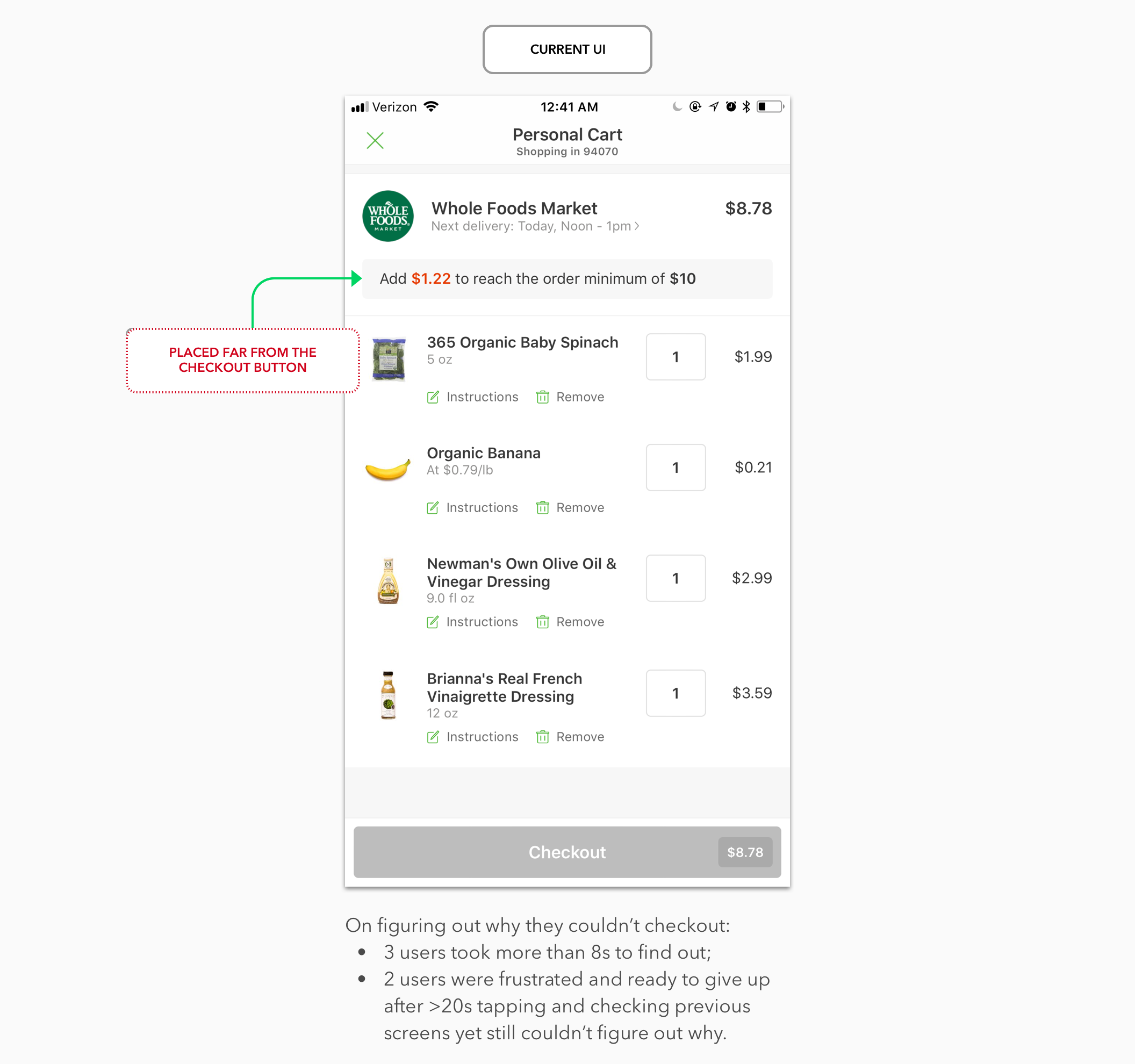**Screenshot Description: Whole Foods Market Cart Page on Mobile Device**

The screenshot captures a Whole Foods Market personal cart page on a mobile device. Here is a detailed breakdown of the elements visible on the screen:

- **Status Bar:**
  - **Signal Strength:** Three out of four cell strength bars.
  - **Carrier:** Verizon.
  - **Wi-Fi Symbol:** Active connection.
  - **Time:** 12:41 AM.
  - **Status Icons:** Moon icon (Do Not Disturb), Power icon, Navigation icon (compass arrow facing upper right), Clock alarm icon, Bluetooth icon, and Battery icon (25% charge, white background with black bar).

- **Top Section Information:**
  - **Upper Left:** Green 'X' to close the cart.
  - **Center Text:** "Personal Cart" in bold.
  - **Subtext:** "Shopping in," followed by "94070" in gray.
  - **Dividing Rectangle:** Gray horizontal divider.

- **Store Information:**
  - **Logo:** Whole Foods Market symbol (green circle with text "Whole Foods").
  - **Text:** "Whole Foods" in black.
  - **Subtext:** "Next delivery today noon-1 PM" in gray.
  - **Cart Value:** "$8.78" in black.

- **Order Information:**
  - **Add to Order:** Gray box with red text "Add" and dollar amount "$1.22" in red.
  - **Minimum Order Requirement:**
    - Green arrow curving towards the right, pointing to the gray box.
    - At the stem of the arrow, a red box with dotted red outline and bold, all-caps red text stating, "Placed far from the checkout button."

- **Cart Items:**
  - **Item 1:** 
    - **Product:** "365 Organic Baby Spinach 5oz Bag"
    - **Quantity:** 1
    - **Price:** $1.99
    - **Icons:** Green instruction icon and green trash can icon with "Remove" text.
  - **Item 2:** 
    - **Product:** "Organic Banana"
    - **Image:** Picture of a banana
    - **Price per Pound:** $0.79
    - **Quantity:** 1
    - **Price:** $0.21
    - **Icons:** Green instruction icon and green trash can icon with "Remove" text.
  - **Item 3:** 
    - **Product:** "Newman’s Own Olive Oil & Vinegar Dressing"
    - **Quantity:** 1
    - **Price:** $2.99
    - **Icons:** Green instruction icon and green trash can icon with "Remove" text.
  - **Item 4:** 
    - **Product:** "Brianna’s Real French Vinaigrette Dressing 12oz"
    - **Quantity:** 1
    - **Price:** $3.59
    - **Icons:** Green instruction icon and green trash can icon with "Remove" text.

- **Footer Section:**
  - **Total Amount Information:**
    - Gray dividing box.
    - Darker gray "Checkout" button with white text "Checkout" and total dollar amount "$8.79" to the right in an even darker gray tone.
  - **Explanatory Text:**
    - Light gray background with detailed user experience issues:
      - First bullet: Indicating that three users took more than 8 seconds to find out.
      - Second bullet: Explaining two users were frustrated and ready to give up after more than 20 seconds of tapping and checking previous screens without understanding why.
      - This descriptive text is situated beneath the screenshot.

In summary, the screenshot effectively captures a cart page from Whole Foods Market, including detailed information on the items in the cart, total amounts, and user interface elements, as well as user experience feedback overlaid on a light gray background.